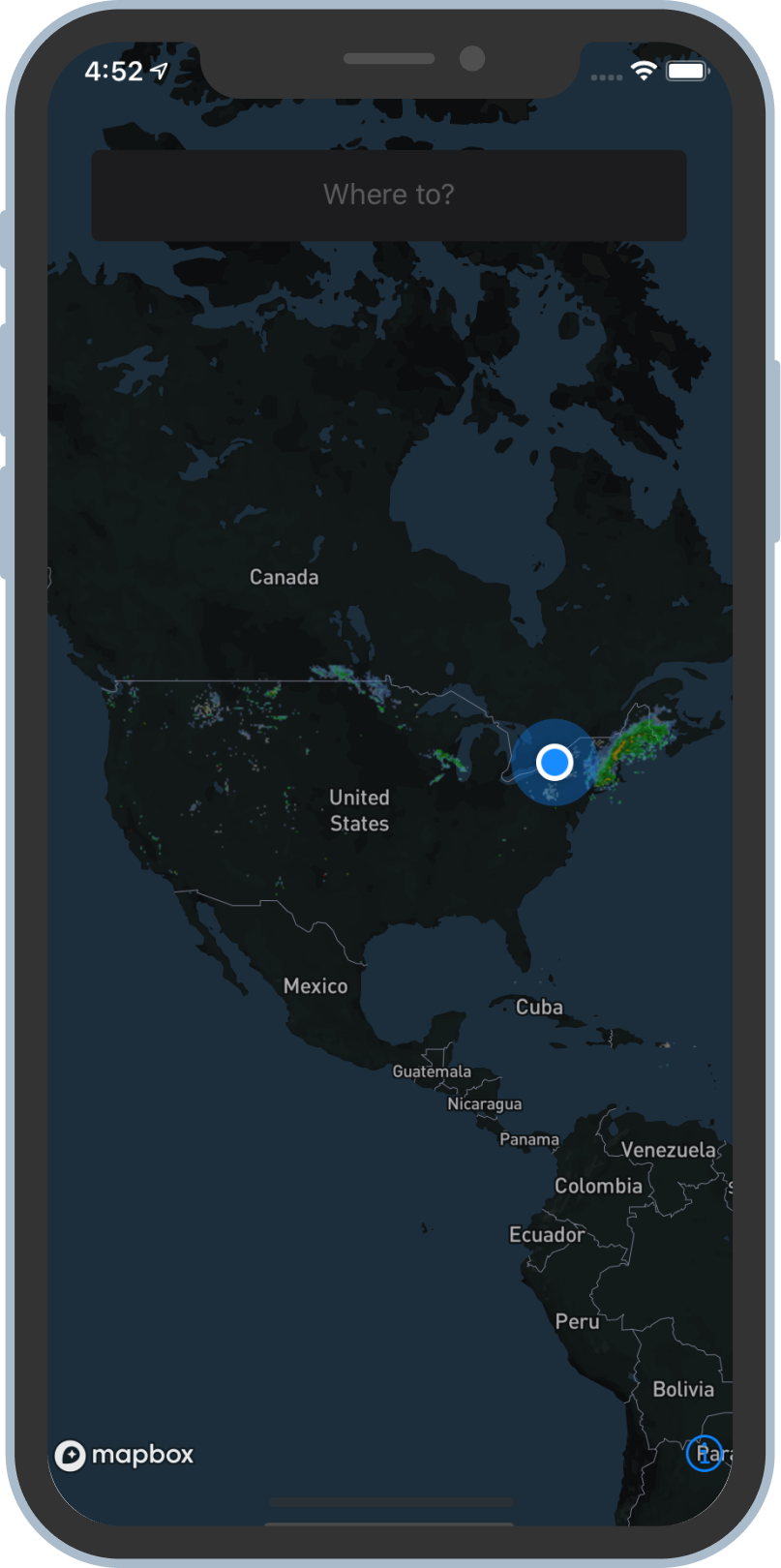This is a screenshot of a geographic map displaying parts of North America and northern South America featuring the United States, Canada, Mexico, Cuba, Guatemala, Nicaragua, Panama, Venezuela, Colombia, Ecuador, Peru, and Bolivia. The map utilizes dark shades of blue, black, and green for a sleek visual presentation. A distinctive blue dot is located in the northeastern United States or possibly the southeastern part of Canada, indicating a specific location of interest. Surrounding the blue dot is a depiction of a weather system, with green and yellow markers signifying an active storm. 

The top section of the screenshot includes a black navigation bar with the text "Where to?" in white, as well as the time display reading "4:52" in the top-left corner. The Mapbox logo is situated in the bottom right-hand corner of the image. Additionally, a blue circle with an eye icon is visible at the bottom of the map, suggesting a feature or setting option. The top right corner of the screen shows standard status indicators including the battery and signal strength icons.